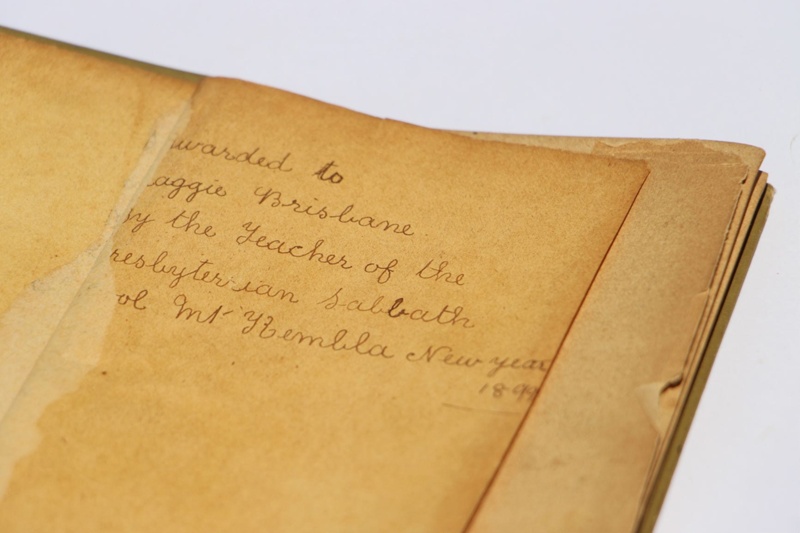This is a detailed photograph of a very old and heavily aged booklet or collection of pages, perhaps an award booklet. The pages are browned with age and have several stains, with some parts torn or missing. The visible writing, which is in cursive, reads "Awarded to Maggie Brisbane by the Teacher of the Year, Presbyterian Sabbath School, Mount Rembla, New York, New Year 1899." The background of the image is a pale gray color, adding contrast to the brown and worn pages. Through the wear and changes in the paper, it's clear this document has historical significance, possibly an accolade or certificate from the late 19th century.